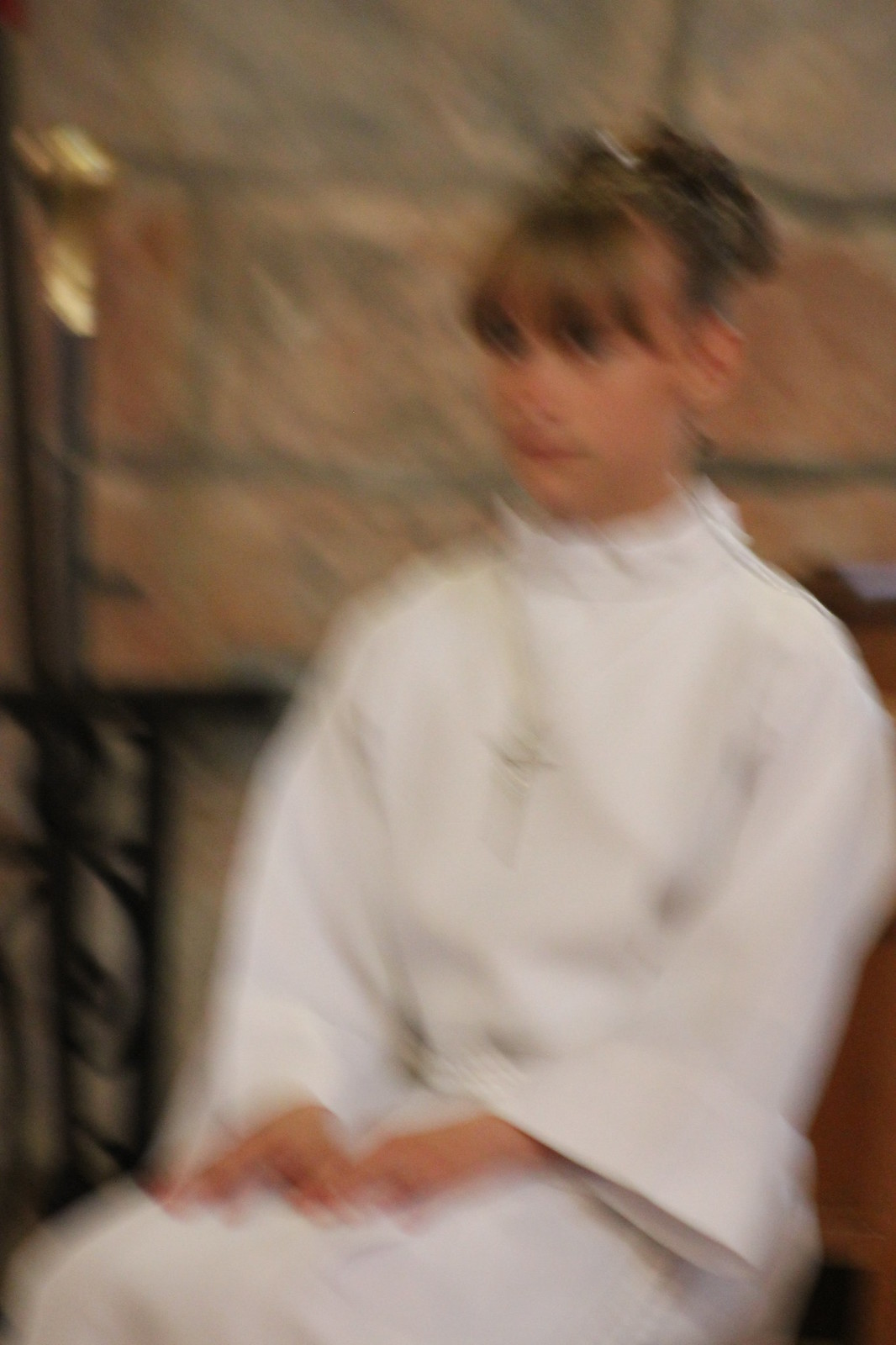The image is a blurry photograph of a solemn-looking young Caucasian woman, seated with her hands resting on her lap. She is dressed in a long, high-necked white garment with three-quarter length sleeves that widen toward the wrists, appearing almost robe-like. Around her neck, she wears a long cross or crucifix. Her hair, a dirty blonde color, is styled up and away from her face, with bangs across her forehead. The woman is positioned facing slightly to the left, allowing a full view of her solemn expression. Behind her is a stone wall made of large, brownish-grey stones with black grout, while to her left stands a wrought-iron staff or post with gold and brass detailing. A black railing is also visible behind her, adding to the image’s setting.